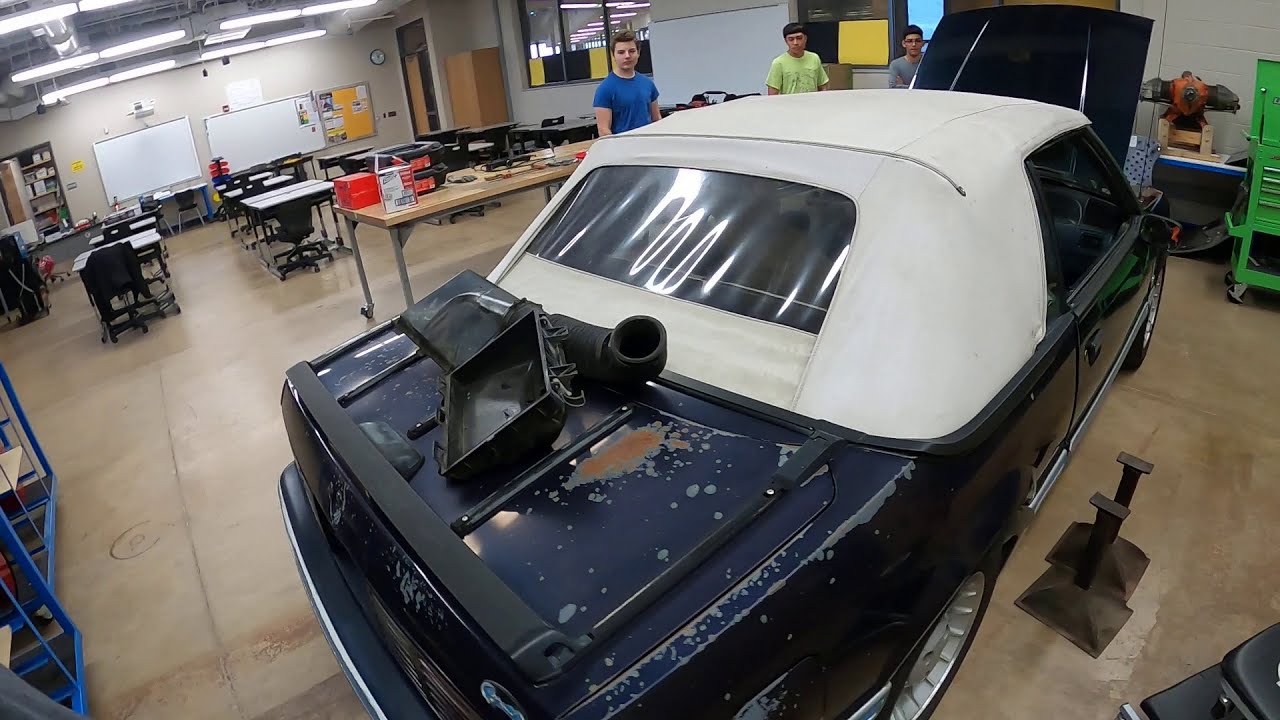The photograph captures a scene inside an auto shop classroom, distinguished by its cement floors and high ceilings with hanging fluorescent lights, emphasizing a well-lit space. Dominating the right side of the image is a large, navy blue car with a white roof and its hood open, revealing the engine bay. The car, showing signs of wear with some rust spots, is parked at an angle facing the top right corner of the frame. 

In front of the car, there are three male students intently observing or working on the vehicle. The students, dressed in a variety of t-shirts—one in blue, one in yellow, and one in gray—appear engaged and focused. To the left of the car, the classroom setup becomes evident with several white desks and rolling chairs neatly arranged, and marker boards affixed to the beige wall. A long wooden table with gray steel legs adds to the workshop's functional layout. Additionally, various auto shop equipment, like jacks, are scattered around, indicative of other ongoing projects or tools in use. The background also reveals windows looking into other parts of the school, adding to the atmosphere of an active, bustling educational environment.